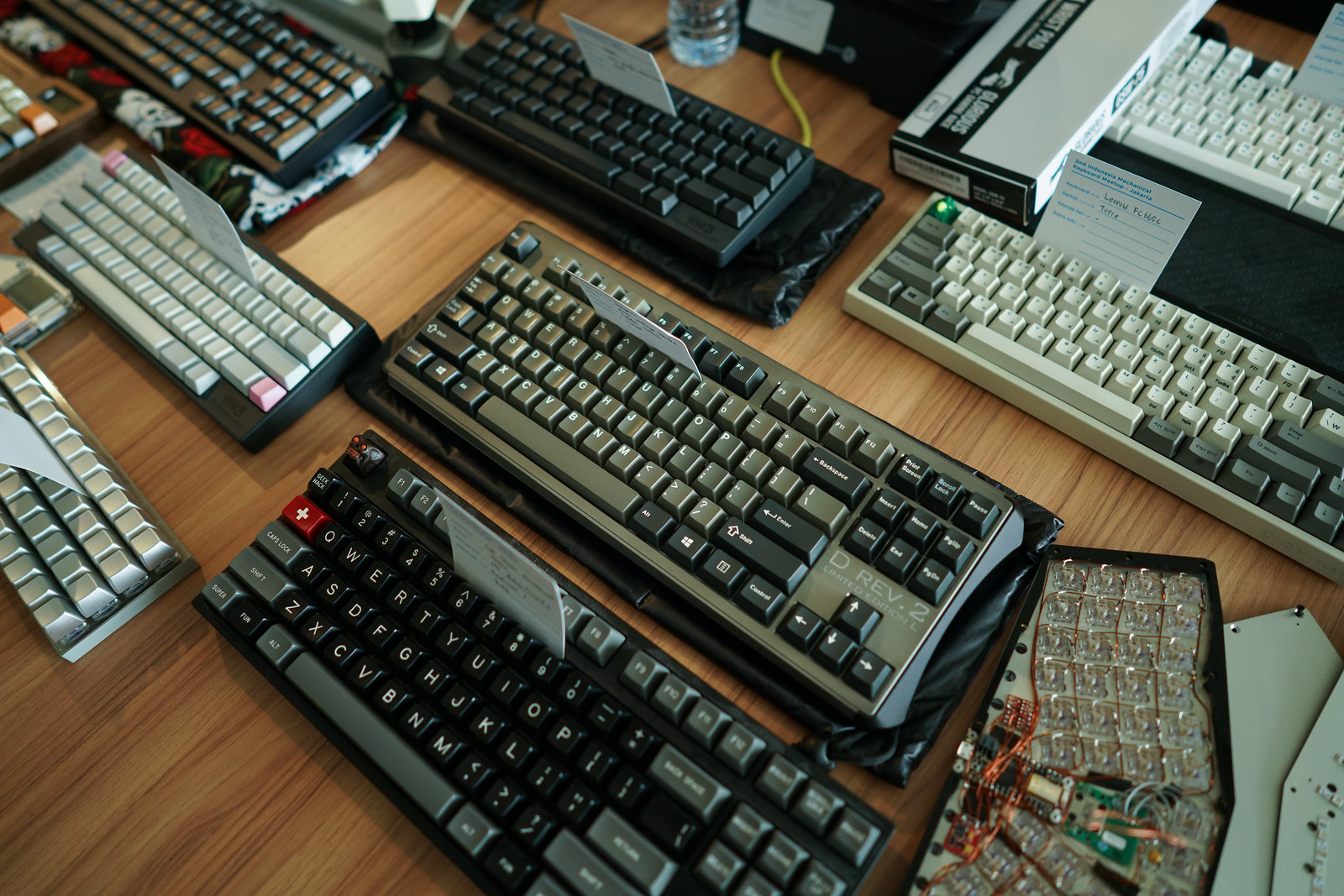A detailed, cohesive caption for the image based on the provided voice descriptions:

This image, a realistic landscape-oriented photograph, showcases approximately 10 computer keyboards arranged diagonally from the top left to the bottom right on a smooth, light brown hardwood floor. The keyboards are a mix of monochromatic hues—black, gray, and white—with white QWERTY letters visible on the keys. Among the keyboards, several exhibit different key functions, including F-keys and number pads, and there are a few with exposed circuitry, suggesting ongoing repairs or customization efforts. Index-like cards are tucked between some keys, likely indicating order numbers or repair details for a custom keyboard business or personal project. In the background, additional tech items like wires and a water bottle are faintly visible, adding context to a workspace setting.